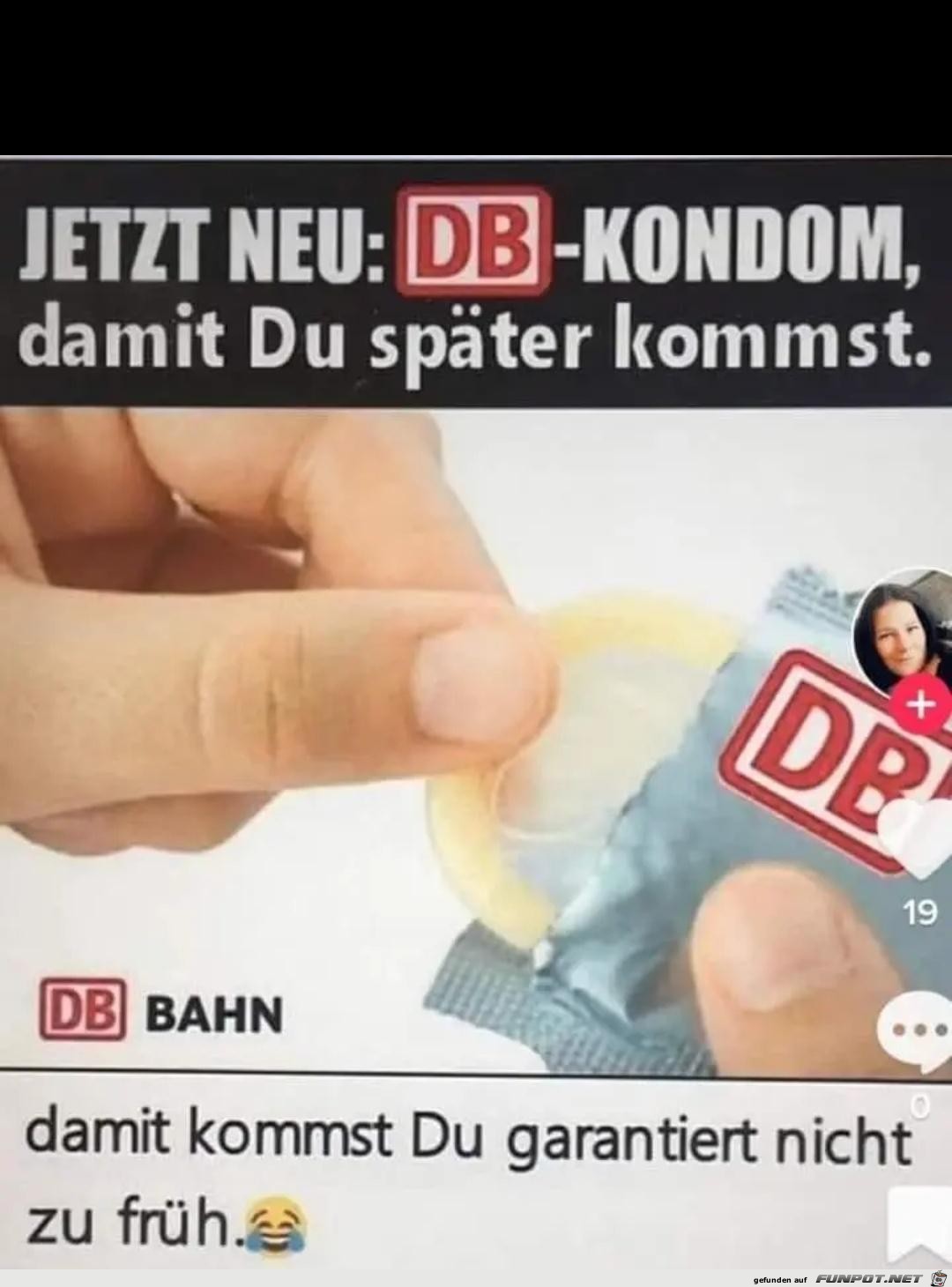This vertically aligned rectangular image resembles an advertisement, potentially a social media post from platforms like Instagram or TikTok. Dominating the top portion of the image is a solid black horizontal rectangular background, followed by a thin gray line stretching from left to right. Below this line, there's a slightly lighter black background displaying text in all caps: "JETZT NEU:" in white or gray letters, and "D-B KONDOM" in red. 

Underneath this, it reads "DAMMIT DU SPEDER KOMPST." The central section features a light gray background where a pair of hands is prominently visible, pulling a condom out of its wrapper. At the bottom, on the same light gray background, the text states, "DAMMIT KOMPST DU GARANTIERT NICHT ZU FRUH," accompanied by a smiley face emoji with tears of joy. Through the text placement and presentation, the image emphasizes safe sex, presenting the information in an engaging, modern, and humorous way.